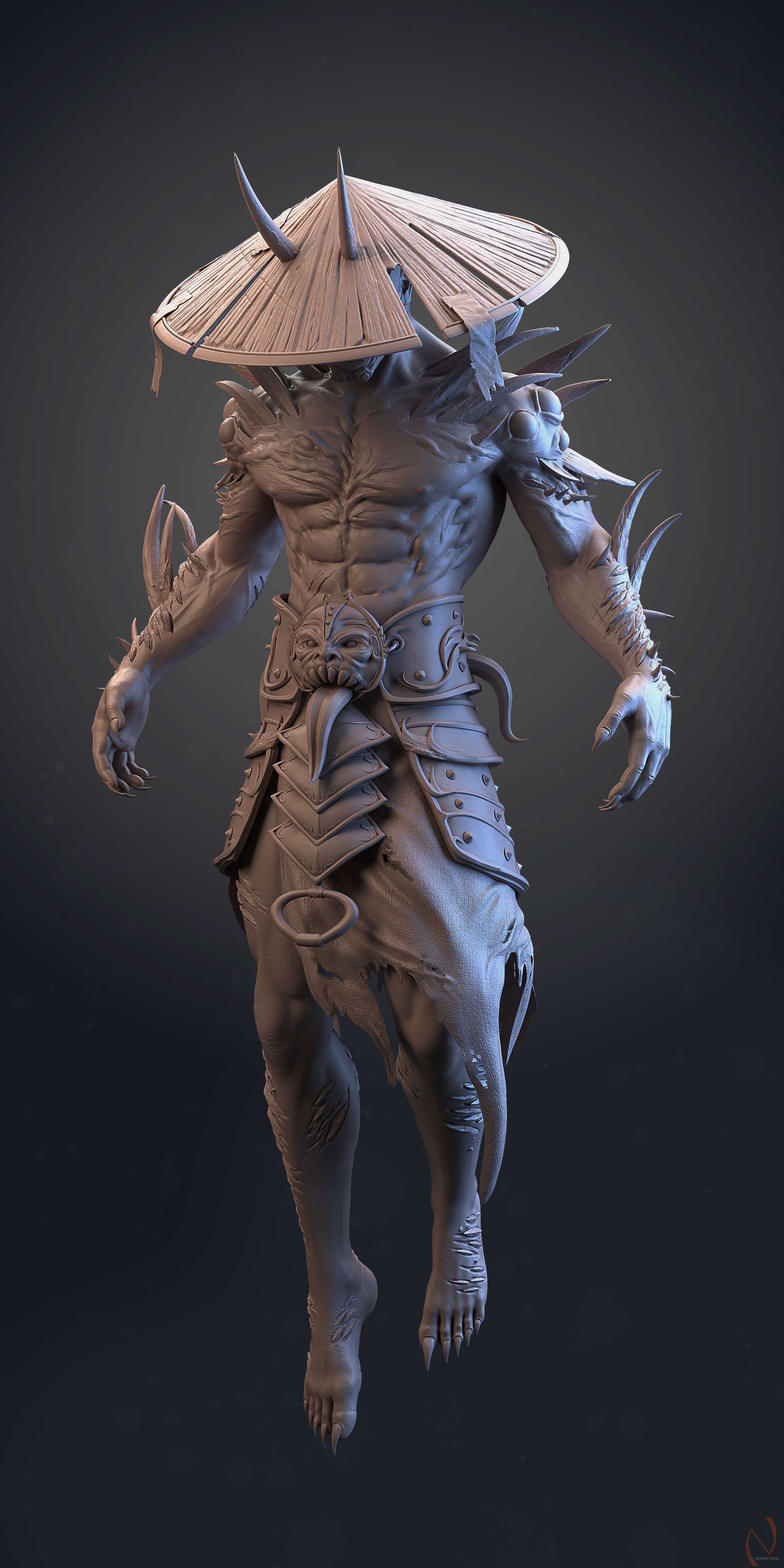The image depicts a detailed 3D model of a video game character or a fictionalized creature designed in a digital modeling program. The character is suspended in midair against a predominantly black background that subtly transitions into whitish, light-gray tones encircling the figure. The creature has a human-shaped, highly muscular body adorned with spikes protruding from its arms and thorns covering various parts. It has a distinctive appearance, featuring a gray, straw samurai hat with two horns protruding through the front. The character’s face is entirely concealed, adding to its mystique. Its attire includes a girdle that prominently displays a dragon-like face with a tongue sticking out. The figure's feet are bare and appear cut, with its legs also displaying similar marks. It has very long, knife-sharp nails, enhancing its menacing presence. The color palette of the character includes fleshy pinks, beige, and subtle blue highlights. This highly detailed model has a formidable and surreal aesthetic, making it seem like a hybrid between a museum artifact and a fantastical game or cinematic character.